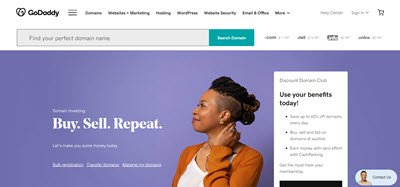This is a detailed cropped screenshot of the GoDaddy homepage. In the top left corner, the GoDaddy logo is prominently displayed. To the right of the logo, a horizontal menu features various categories, followed by a "Free Offer" section, a "Log In" option, and a shopping cart icon at the far end. Just below this menu, a search bar is positioned for user queries, accompanied by logos of businesses that utilize GoDaddy services to its right.

The bottom section of the webpage is set against a striking purple background. Centrally, there is an image of a woman. To her left, the text "Buy, Sell, Repeat" is displayed, highlighting some features in small white letters beneath it. On the right side, the phrase "Use your benefits today" is written inside a white rectangular box, with an actionable button situated just below. In the bottom right corner, a chat bubble icon indicates the option to speak with a customer service representative. The webpage header is in white, while the main body of the webpage features a photo backdrop with the purple theme seamlessly transitioning into it.